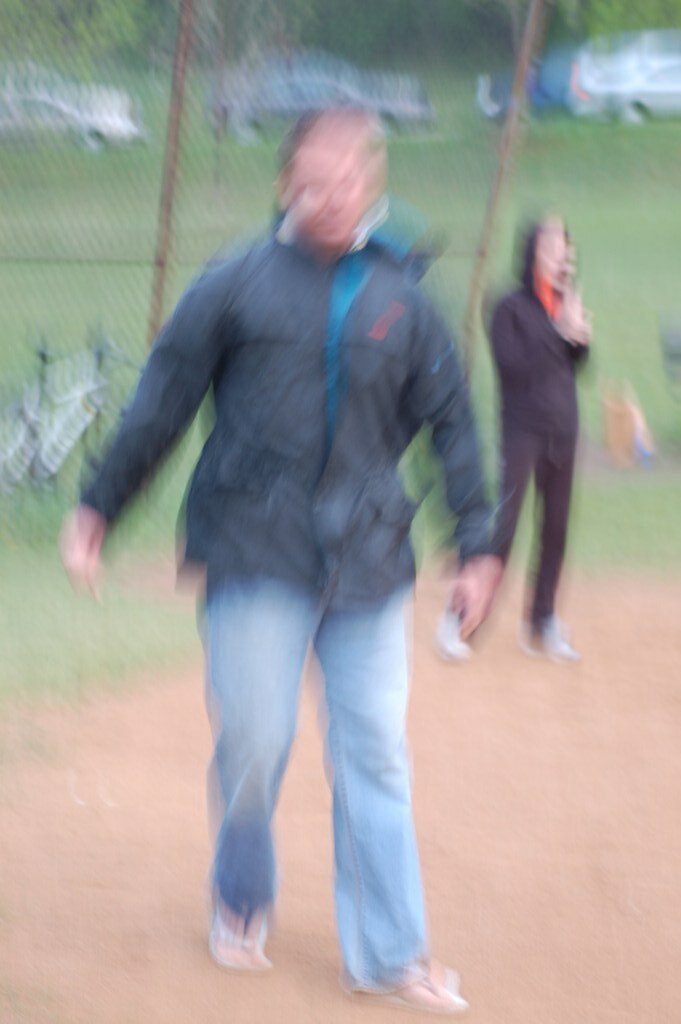In a blurred photograph, the foreground features a sandy area where a person stands, dressed in a black jacket, blue jeans, and tennis shoes. Adjacent to them, another individual is seen standing, cloaked in a black hooded jacket and matching black pants. Surrounding this sandy spot is a grassy expanse punctuated by parked bicycles. In the background, numerous cars are visible alongside tall utility posts. Scattered within this scene, various toys are noticeable, adding a touch of playfulness to the otherwise serene setting.